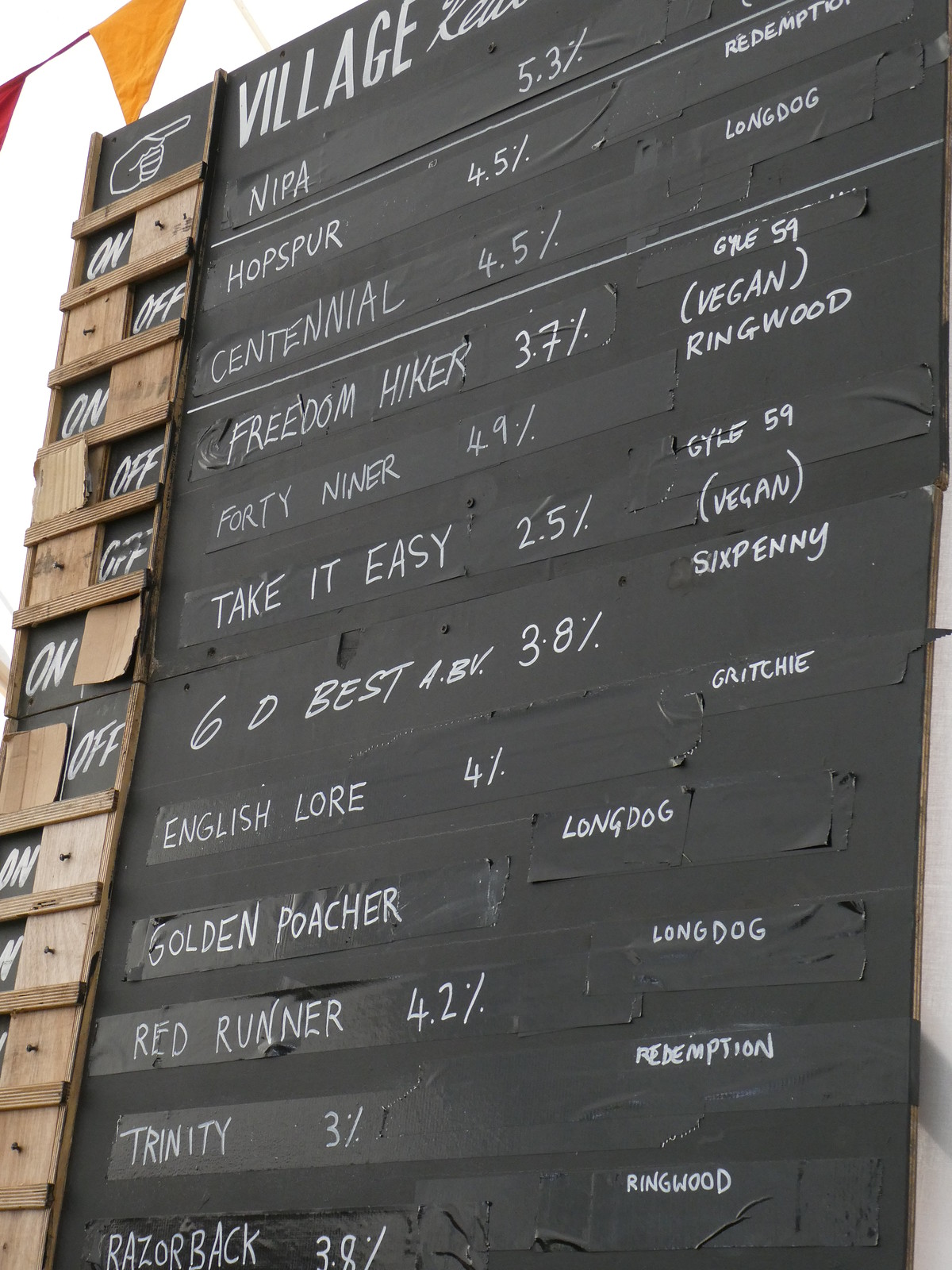This photograph features a sign resembling a chalkboard with a black background and white lettering. The top of the sign partially reads "village," but the full title is cut off due to the photo's framing. Below the title, there is a detailed list of names accompanied by percentages. The list includes: Nipa (5.3%), Hobser (4.5%), Centennial (4.5%), Freedom Hiker (3.7%), 49er (4.9%), Take It Easy (2.5%), GED Best (3.8%), English (4.4%), Golden Roach (blank), Red Runner (4.2%), Trinity (3.0%), and more, though the lower portion of the list is also cut off.

The left side of the sign features wooden slots that can slide horizontally, marked with "on" and "off" depending on their position. These details are written in what appears to be a style mimicking hand-written chalk on a classroom chalkboard. The background above the sign is described as very white, and there is a yellow flag visible in the top part of the photograph.